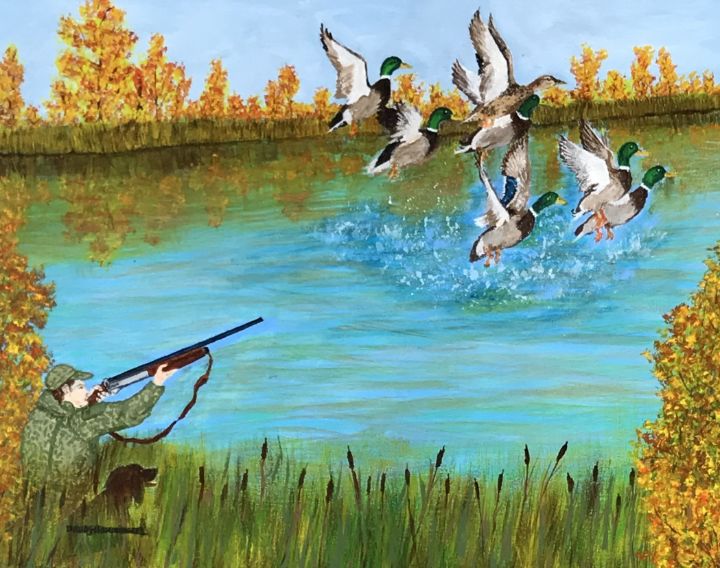The illustration is a vivid watercolor scene of a duck hunting expedition in autumn. The background is dominated by a blue sky and vibrant orange trees, their colors reflecting in a greenish-blue lake. Central to the image are seven or eight mallard ducks, characterized by their green heads, yellow beaks, dark brown chests, gray bottoms, white undersides of their wings, and orange feet, frantically taking flight from the water. Among them is a unique duck colored in shades of brown, distinguishable from the rest. In the bottom left, a man dressed in full camouflage gear, with a matching hat, stands poised behind tall green reeds, his rifle aimed at the sky. Beside him, a black Labrador retriever intently watches the ducks, ready to retrieve any that are shot. The scene is rich with details of foliage and water lilies, capturing the essence of a tranquil yet dynamic hunt in the crisp autumn air.